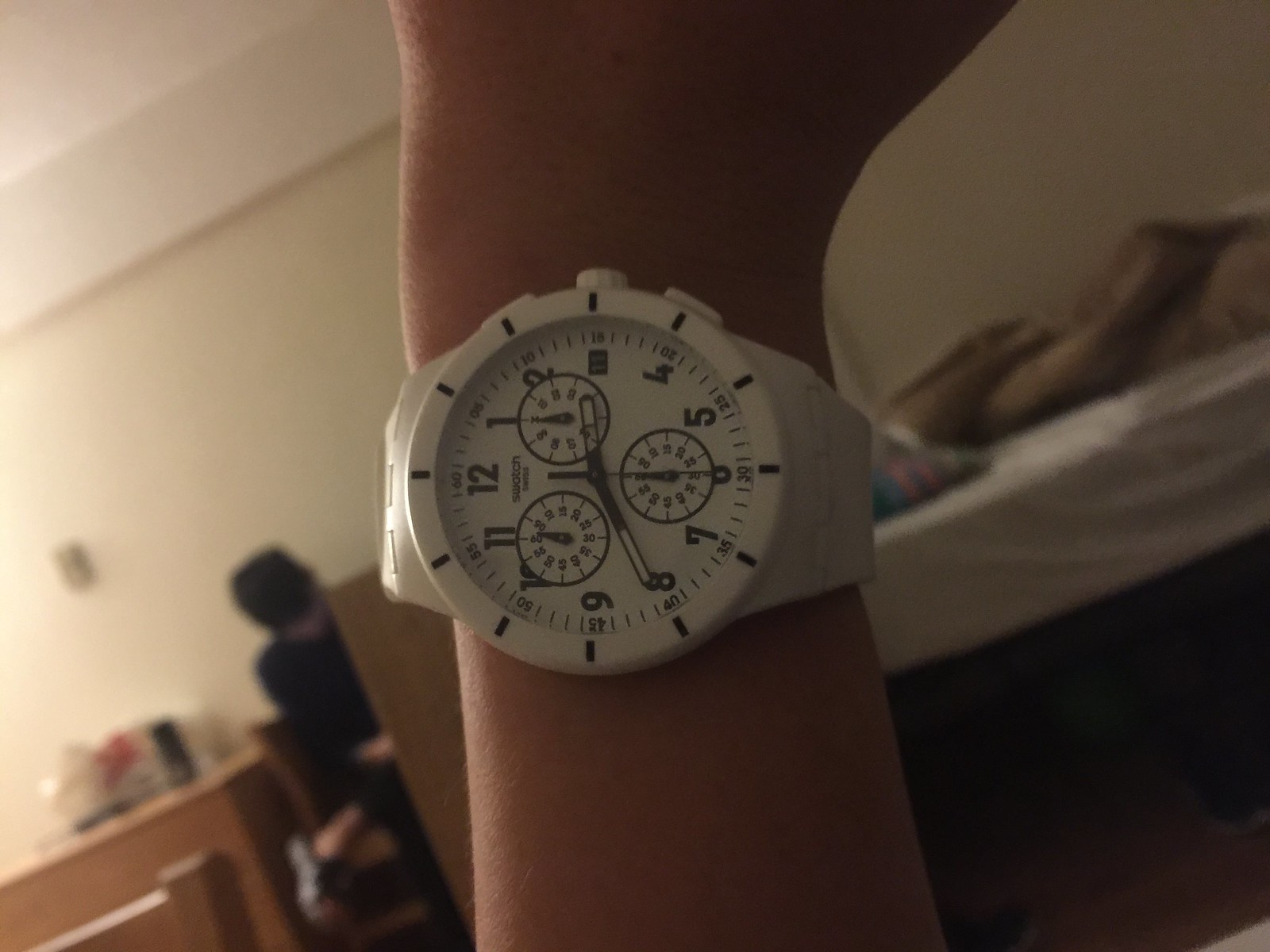The image depicts a close-up of the hand of a Caucasian individual wearing a white Swatch analog wristwatch. The watch features a pristine white face with bold black numbers ranging from 1 to 12, as well as smaller markings for each second, in increments of five, encircling the dial. The watch also includes three smaller sub-dials integrated within the main face, each displaying different times with their own sets of black numbers and hands. Prominently, the hour hand is pointing towards the 3 (positioned at the top of the watch), the minute hand is at the 8 (bottom right), and the thin second hand is directed towards the 6 (right side). The brand name "Swatch" is inscribed in black along the top left arc of the watch. The watch’s white buttons and a white wristband complement its clean design. In the background, on the right side, there is a bed adorned with a white cover, a brown cover, and a colorful blue and red pillow. A person dressed in all black is visible on the left of the image, sitting with one leg crossed over the other, beside a cabinet.